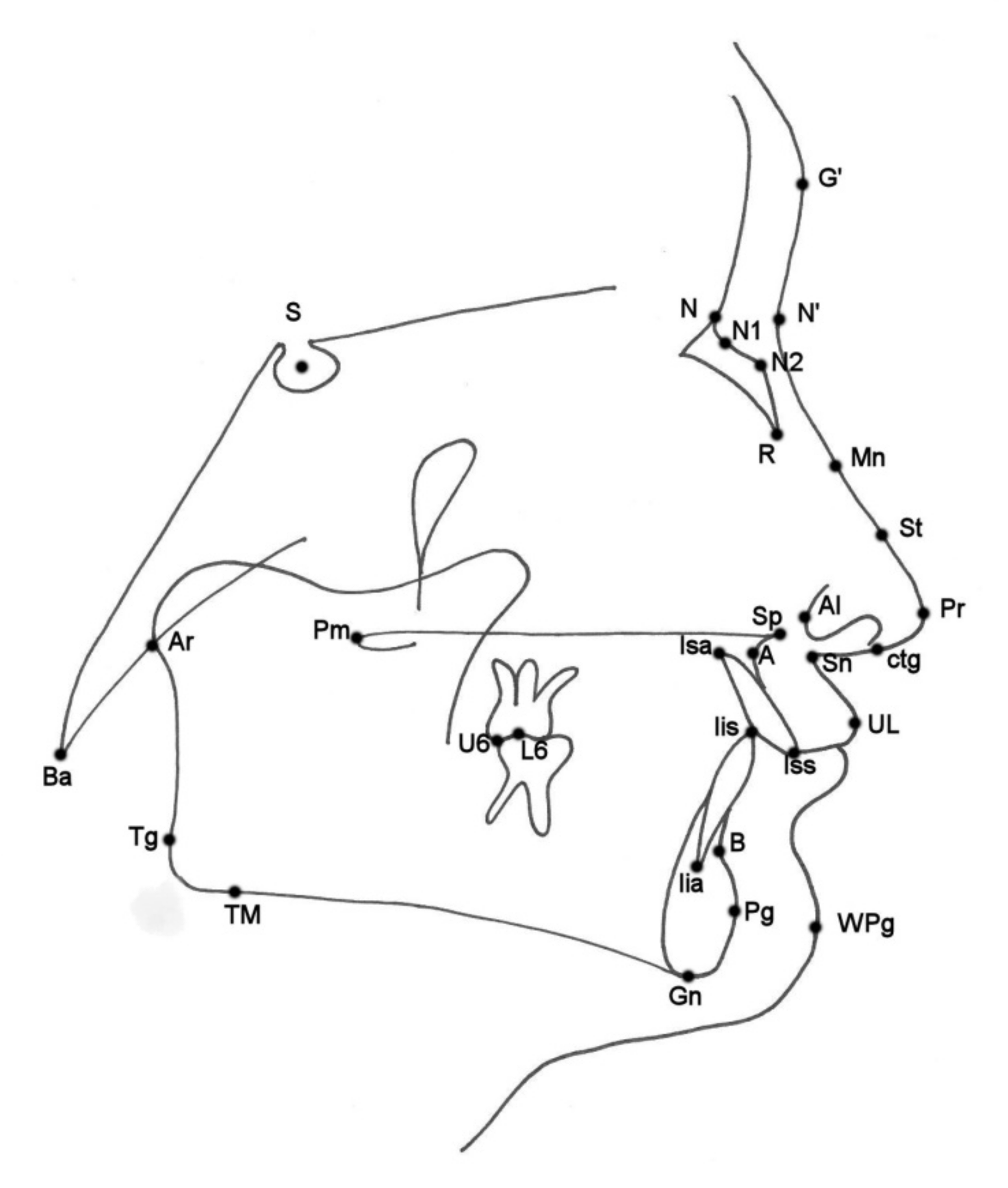This image is a complex, abstract diagram resembling a connect-the-dots puzzle. Instead of numbers, it utilizes an assortment of letters and symbols to guide the connections. Featured prominently are black dots on various lines, creating an intricate web of squiggly lines. The letters include sequences such as AR, BA, TG, TM, GN, PG, WPG, UL, CTG, PR, AI, SP, SH, LIA, LSS, along with symbols like '1', 'G', 'PM', 'U6', 'L6' and more. This pattern suggests constructing a recognizable shape—potentially a face—similar to how one would draw by connecting numbered dots. Notably, the diagram includes what could be interpreted as facial details, such as the outline, a few teeth, and minimalistic representations of eyes. This blend of letters and lines forms a detailed and slightly chaotic visual, inviting viewers to decode its hidden structure.